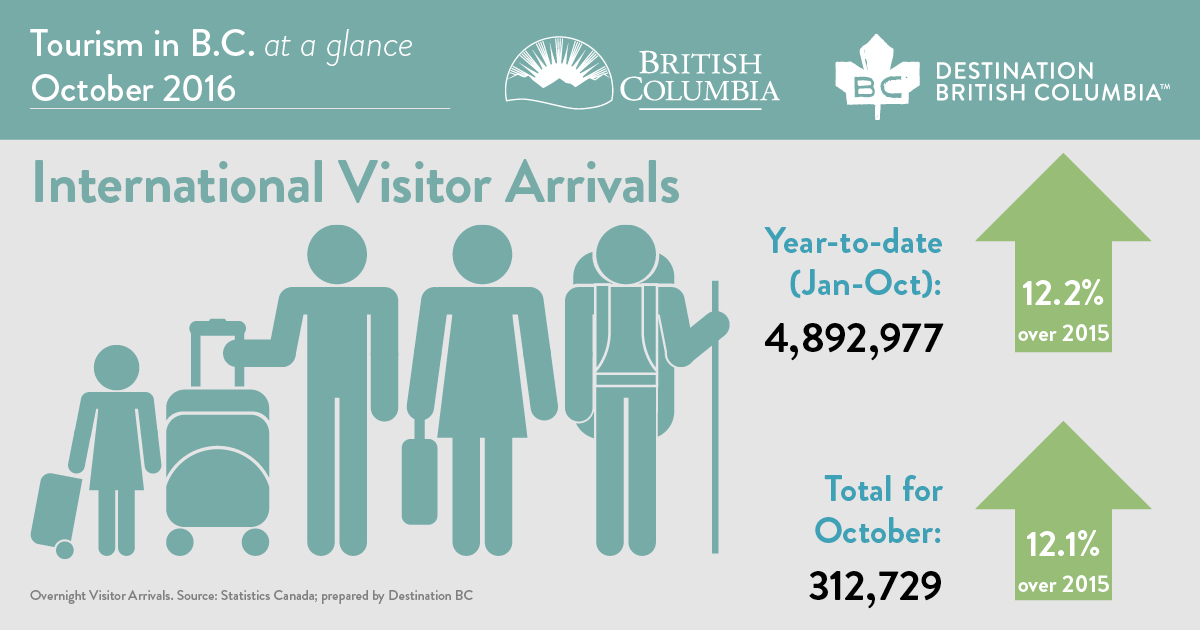The image is a detailed data visualization poster for British Columbia tourism, titled "Tourism in BC at a Glance, October 2016." The top section features a blue-gray background with white text, displaying logos for British Columbia and Destination British Columbia. There's an image of a sunrise over mountains and a maple leaf with the initials "BC." 

The bottom section transitions to a light gray background with teal, blue, black, and white text. This part is dedicated to "International Visitor Arrivals" and includes stick figure illustrations of travelers—a family with children wheeling suitcases, adults carrying briefcases, and a male hiker with a backpack and walking stick. 

On the right side, it notes the "Year to Date" visitor count as 4,892,977 from January to October, marked by a green arrow indicating a 12.2% increase over 2015. For October alone, the visitor count is 312,729, with an upward arrow highlighting a 12.1% rise compared to 2015. The lower left corner features a legend clarifying these as "Overnight Visitor Arrivals," sourced from Statistics Canada and prepared by Destination BC.